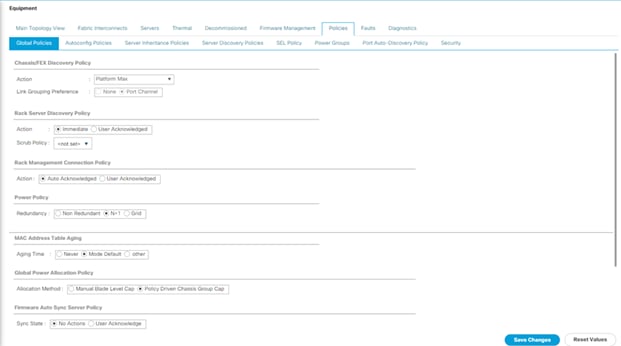The image depicts a screenshot from an application interface showcasing several headings across the top of the screen. The headings, although somewhat difficult to read due to small font size and poor image clarity, appear to include "Equipment," "Main Topology View," "Future Improvements," "Services," "Management," and "Policies," among others. The visible interface mainly focuses on the "Policies" tab, which is currently selected.

On the left-hand side of the screen, there is a menu presenting various settings. These settings are accessible through radio buttons and pull-down menus. The radio buttons allow the user to select one option among a set; for instance, under the "Action" category, two specific options are available for selection. In other cases, options may come in groups of three. The interface provides a comprehensive view of how policies can be managed, offering a structured layout of configurable settings predominantly featuring radio button selections.